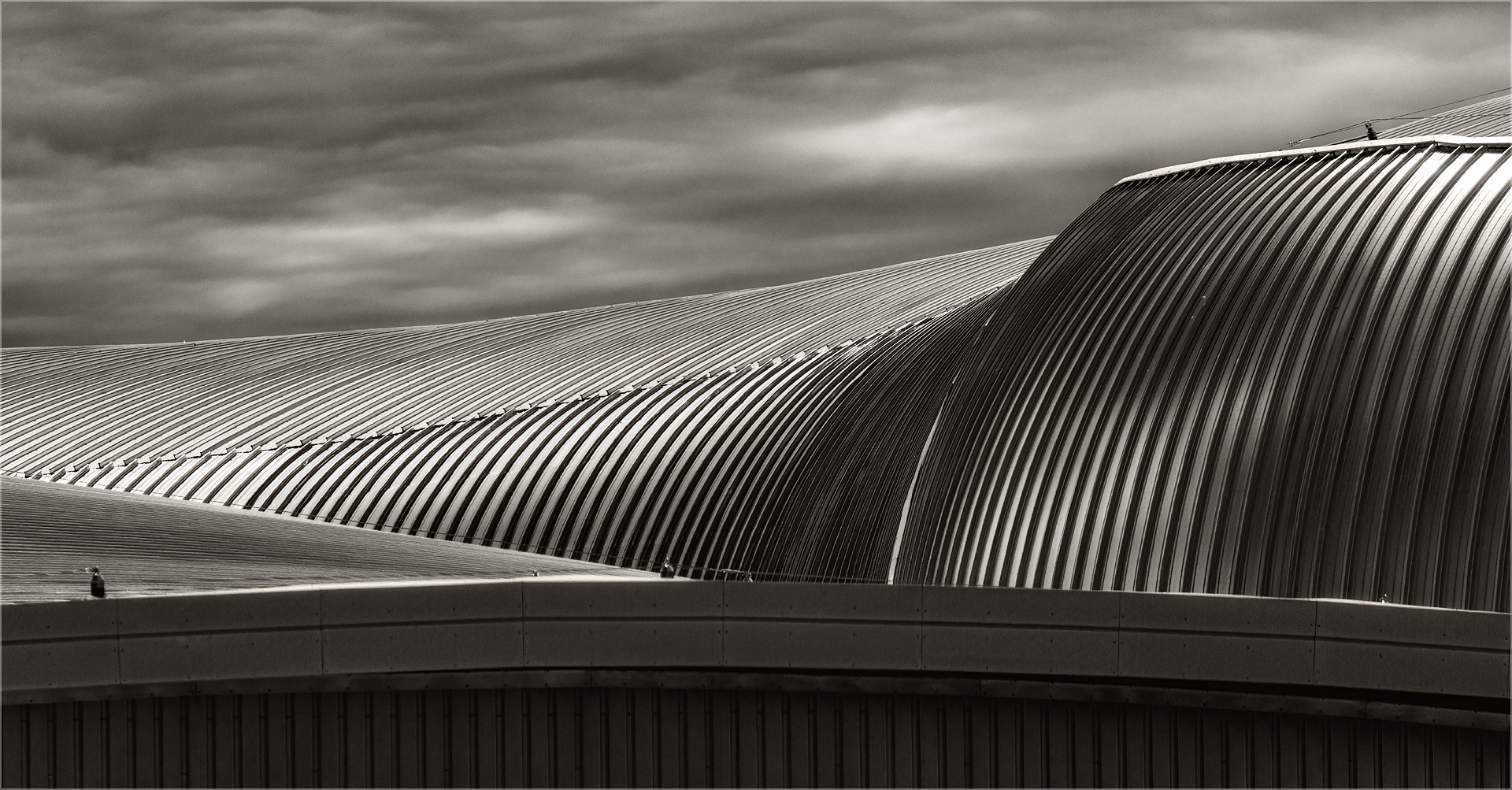This black-and-white image features an abstract, distorted view of what appears to be a large metal building. The structure, reminiscent of the World Trade Center or a stadium roof, is characterized by numerous vertical and curved lines that give it a wavy, bending appearance. The sky above is densely clouded, creating a gloomy and oppressive atmosphere with dark, stormy clouds. The building, adorned with horizontal and vertical stripes, is made of metal, enhancing its modern and industrial look. The image, which also includes indistinct shapes that might be people or birds atop the building, captures a scene that is both intriguing and somewhat unsettling due to its surreal, almost optical illusion-like quality.